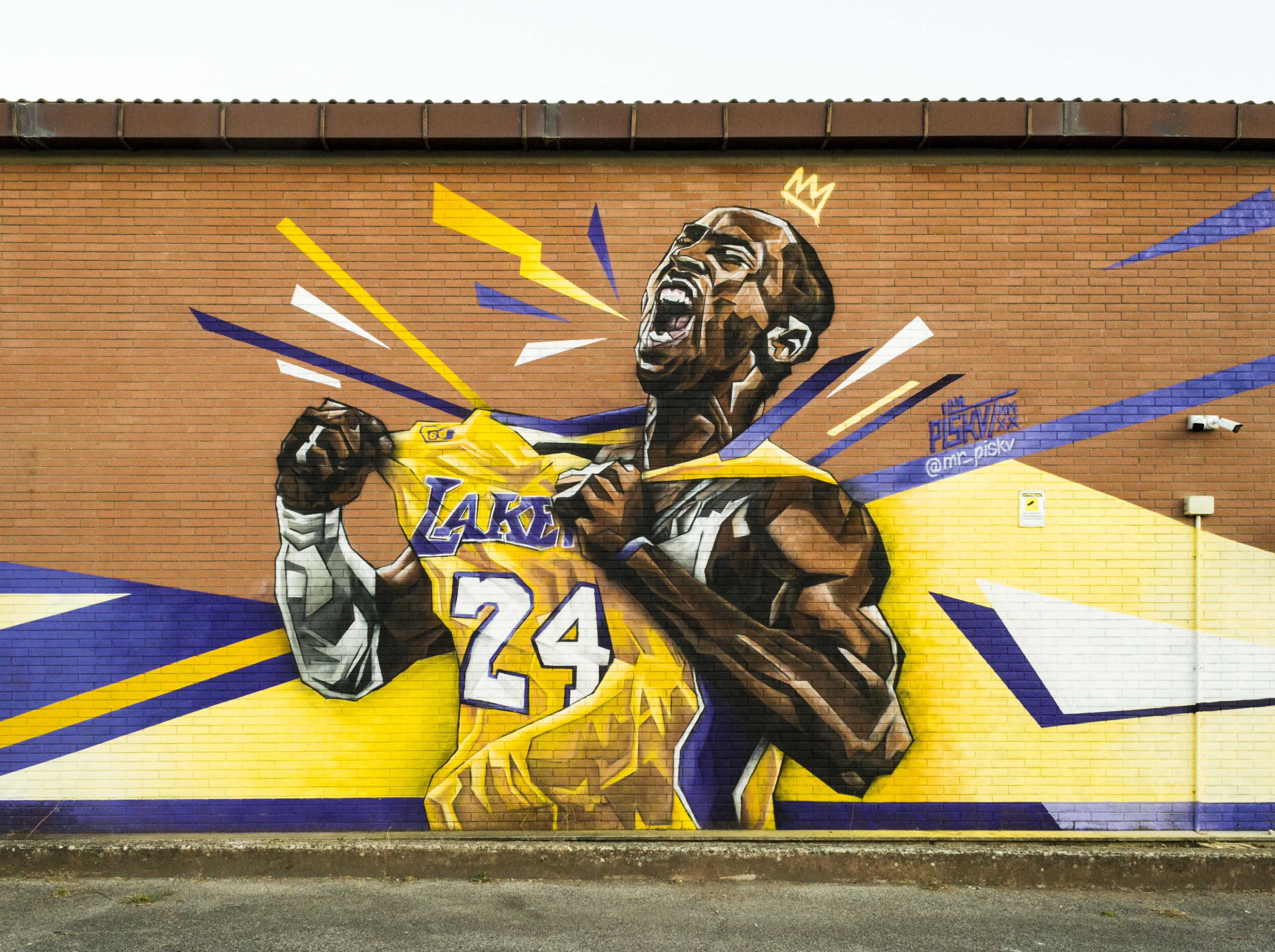This image features a large, striking mural painted on the side of a brick building, likely a school, given the presence of security cameras and a sidewalk with no visible doors or windows. The mural vividly depicts Kobe Bryant, the legendary Los Angeles Lakers player, identifiable by the iconic number 24 on his yellow Lakers jersey, which also exhibits hints of purple and white. 

The artwork captures Kobe mid-celebration, his eyes closed and mouth open as he pulls on his jersey, exuding a sense of triumph and intense emotion. Above his head, a simple crown is painted, signaling his "King" status in the world of basketball, although the crown appears less refined compared to the rest of the mural. The background complements his jersey with abstract geometric patterns in Lakers' colors: gold, purple, and white, enhancing the dynamic and vibrant feel of the piece. 

Additionally, the artist's social media handle, @MrPiskey, is inscribed nearby, attributing the work to them. Overall, this mural is a powerful tribute to Kobe Bryant, blending both realistic portraiture and abstract design to celebrate his legacy.